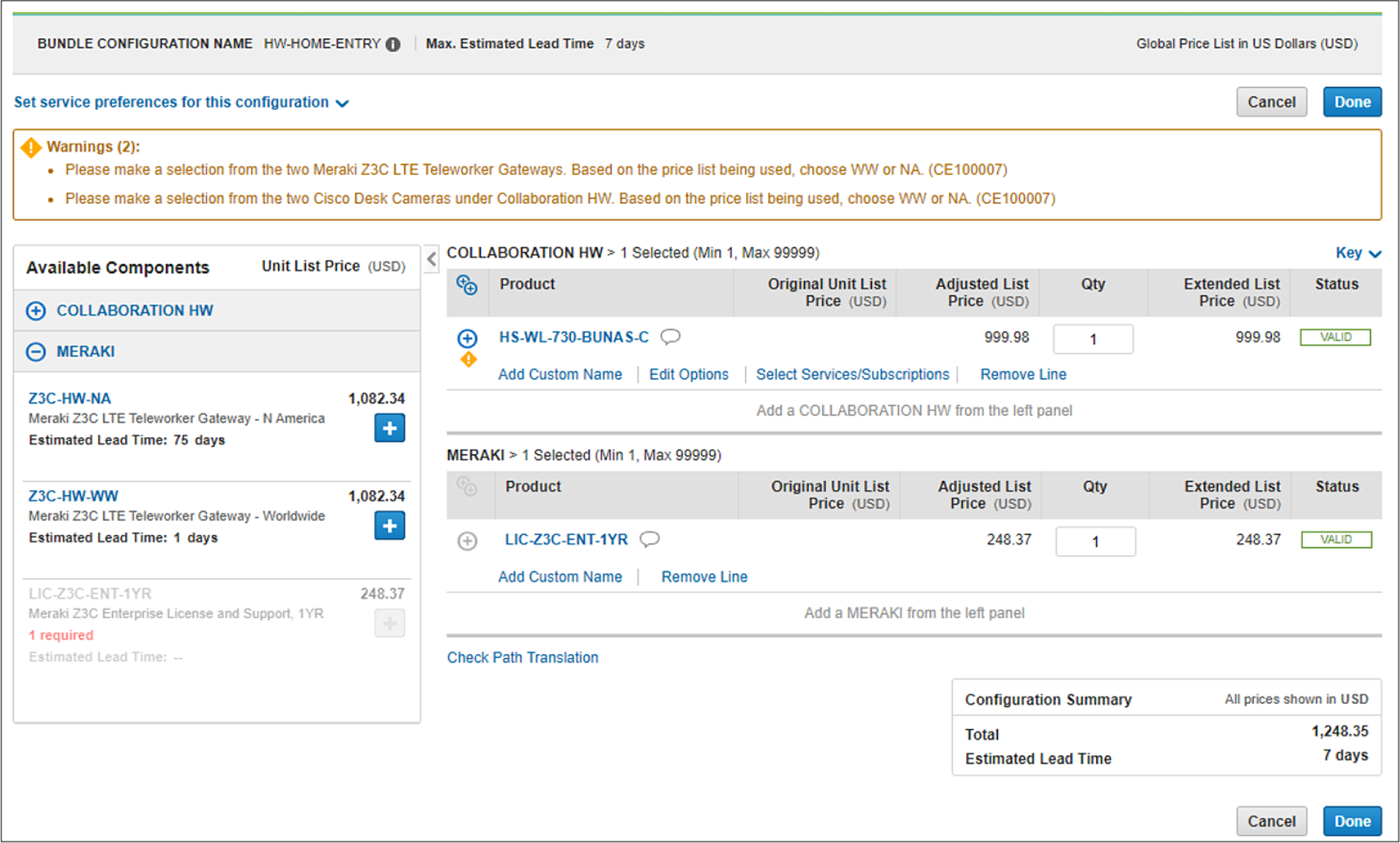**Descriptive Caption:**

The image displays a detailed configuration and pricing interface for telecommunications hardware. At the top, there's a gray bar labeled with a bundle configuration name, "HW to Home Entry." This section estimates a maximum lead time of 7 days for the hardware, with the global price visible upon request. Below, a blue section instructs users to "Set Service Premises for This Configuration," offering "Cancel" and "Done" options.

A prominent yellow box beneath highlights two critical warnings associated with Meraki ZDC LTE teleworker gateways. These gateways must be selected based on price, with options for "Worldwide (WW)" or "North America (NA)" configurations. The reference code "T10007" is given for making selections for two Cisco desk cameras under the collaboration hardware category, which follows the same price-based selection criteria (WW or NA).

The available components section lists detailed pricing:
- Collaboration HW
- Meraki ZDC-HW-NA (North America): Meraki ZDC LTE teleworker gateway with an estimated lead time of 7 days, priced at $1,082.34.
- Meraki ZDC LTE teleworker gateway (Worldwide): HS-WL-L30-BNUS-C priced at $999.98, with an additional license component labeled LIC-C3C-TNT-1YR.

Each component clearly displays the net list price and associated details, ensuring users can make informed purchasing decisions based on regional and pricing preferences.